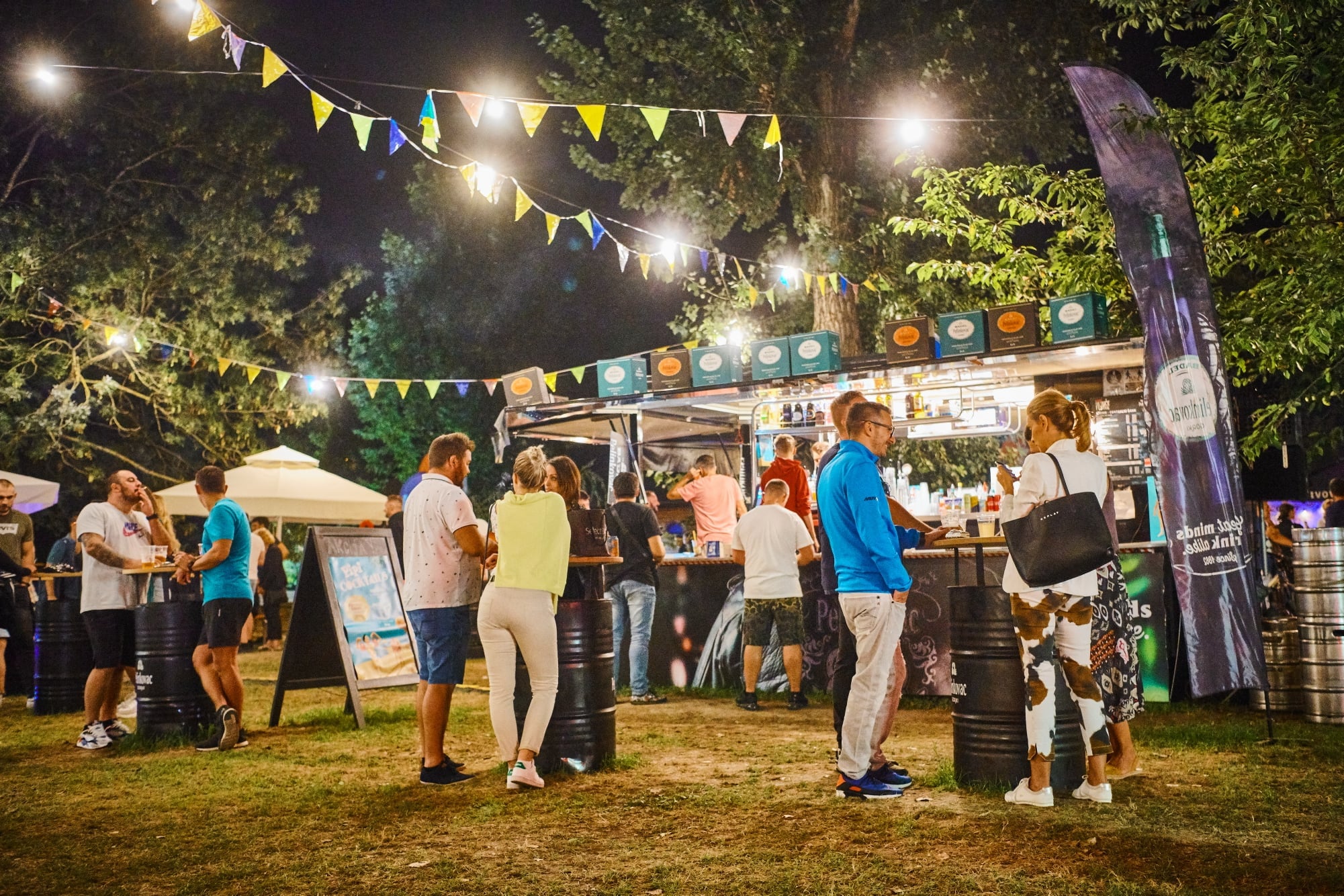The image captures a vibrant night gathering around a food vendor scene, set against a backdrop of trees adorned with yellow and blue pennants strung overhead, interspersed with lights creating a festive atmosphere. The people, dressed in a mix of formal and casual attire, are standing on a small lawn, engaging in conversation around black barrels repurposed as tables. The focal point is a food truck with a wide-open bar area and visible signage, serving enthusiastic patrons. A tall, dark vertical banner marks the right end of the vendor site, while a beige-canopied area to the left houses several more attendees. The scene exudes a spirited communal ambiance under the dark sky lit by artificial lights, showcasing a blend of social interaction and culinary delight.